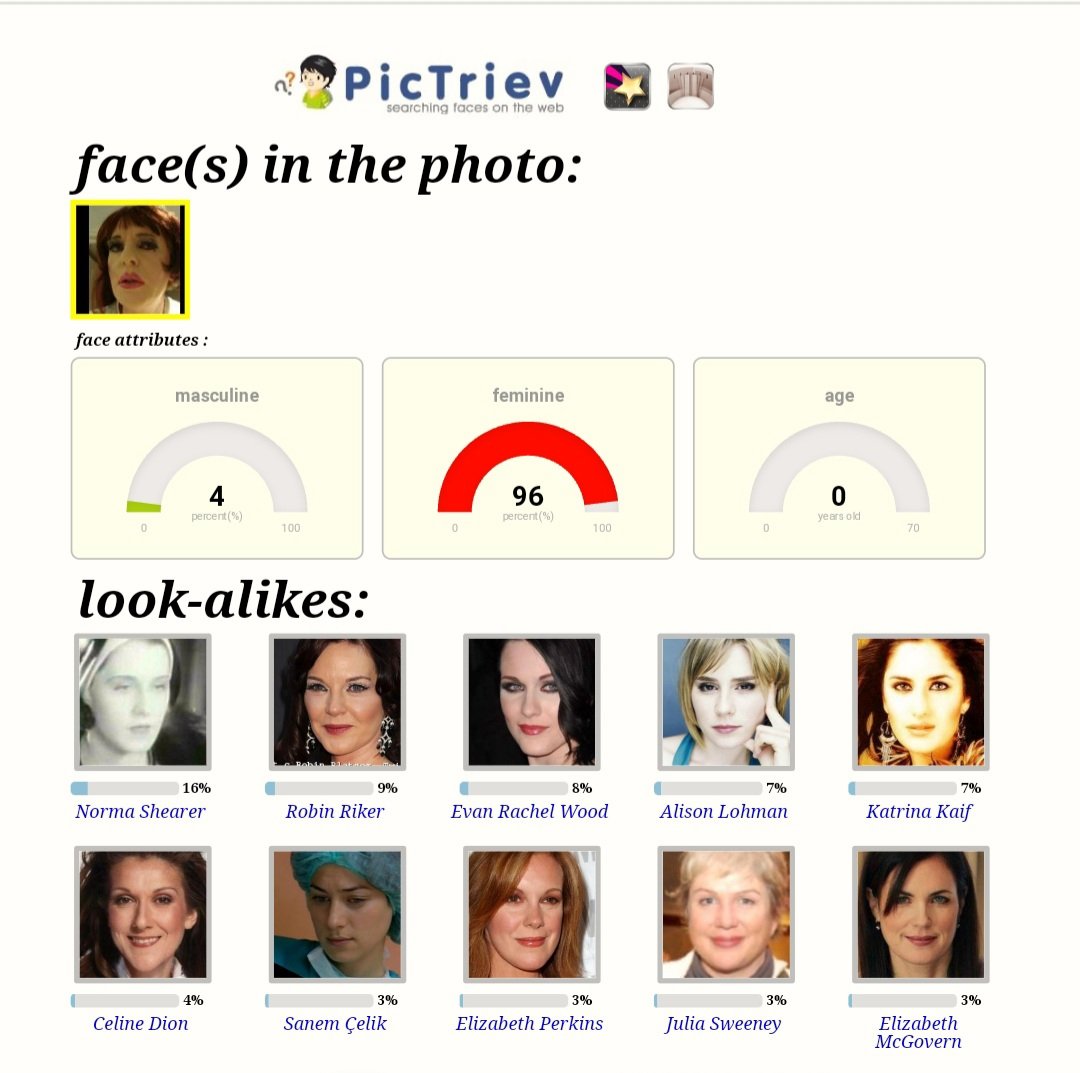The image is titled "PICTRIEV: Searching for Faces on the Web" and prominently features various elements that analyze and compare a face within a photo. At the top, "PICTRIEV" is spelled out, followed by the description, "Searching for Faces on the Web." Below, it reads "Face(s) in the photo," highlighting a white woman's face adorned with noticeable lipstick, enclosed in a yellow box. 

On the left side of this main face picture, there is a section labeled "Face Attributes," presenting three beige semicircular gauges resembling speedometers. These gauges score different attributes: the first shows "Masculine: 4," the second "Feminine: 96," and the third indicates "Age: 0," suggesting no age determination was made.

Beneath the face attributes section, there's a "Lookalikes" area featuring ten smaller images of various women, arranged in two rows, each with a corresponding similarity percentage. The women include Norma Shearer (16%), Robin Riker (9%), Evan Rachel Wood (8%), Allison Lohman (7%), Katrina Kaif (7%), Celine Dion (4%), Sanam Saeed (3%), Elizabeth Perkins (3%), Julia Sweeney (3%), and Elizabeth McGovern (3%). This image appears to be from a website designed to analyze facial characteristics and suggest celebrity lookalikes based on the input photo.